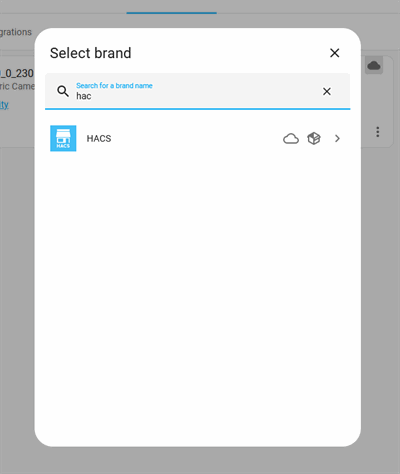The image is a heavily cropped screenshot taken from a website or software application, focusing on a specific feature. The screenshot showcases a white pop-up box with a translucent background, making the underlying interface barely visible. The pop-up contains the title "Select Brand." Below the title is a search bar with a blue placeholder text that reads, "Search for a brand name." The user has searched for the term "HAC," yielding a single result for a brand named "HACS." The brand's logo is a blue square with a white house-like shape inside it. Adjacent to the search results are three icons: a cloud, an open box, and a right-facing arrow. These icons likely indicate different actions or statuses related to the brand search result.